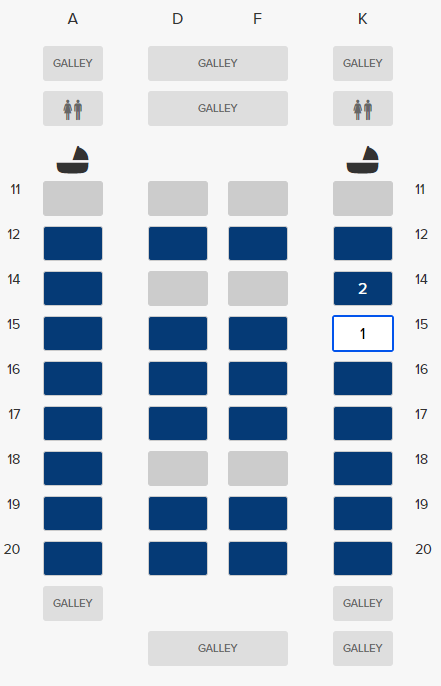This image is a vertically-oriented diagram illustrating a seating arrangement, likely on a boat. The background is a medium gray tone, providing contrast to the various elements displayed.

At the top of the image, there are black letters: "A", "D" and "F" positioned close to each other, followed by "K". Directly beneath the letter "A" is a gray box labeled "galley". Below this, another gray box features icons representing a man and a woman. 

A depiction of a black boat is situated further down, above a series of numbered rectangular boxes from 11 to 20. The box labeled 11 is grayed out, while boxes 12 through 20 are filled with navy blue, signifying occupied or available spaces. Beneath the box labeled 20 is another gray box marked "galley".

Reappearing at the top are the letters "D" and "F". Below them are two elongated gray boxes, each labeled "galley". The number 11 appears again, grayed out, followed by a box labeled 12 in navy blue. This sequence of alternating navy blue and gray boxes continues with numbers 14, 15, 16, 17, 18, 19, and 20, indicating different seat statuses.

Finally, under the letter "K" at the top, there is another annotated gray box marked "galley" with a man and woman icon below, followed by the boat image. This section mirrors the earlier pattern, with numbered boxes 11 through 20 showing a mix of grayed-out and navy blue fill. Unique boxes labeled 14 and 15 highlight white numbers "2" and "1" respectively, enclosed in light blue borders. The remaining boxes, 16 through 20, are navy blue.

Concluding the image are two more gray boxes labeled "galley" underneath the number 20, maintaining the structured layout throughout the diagram. The overall design seems to represent seating zones, possibly within a large cabin or deck area of the boat, clearly demarking various areas and facilities.